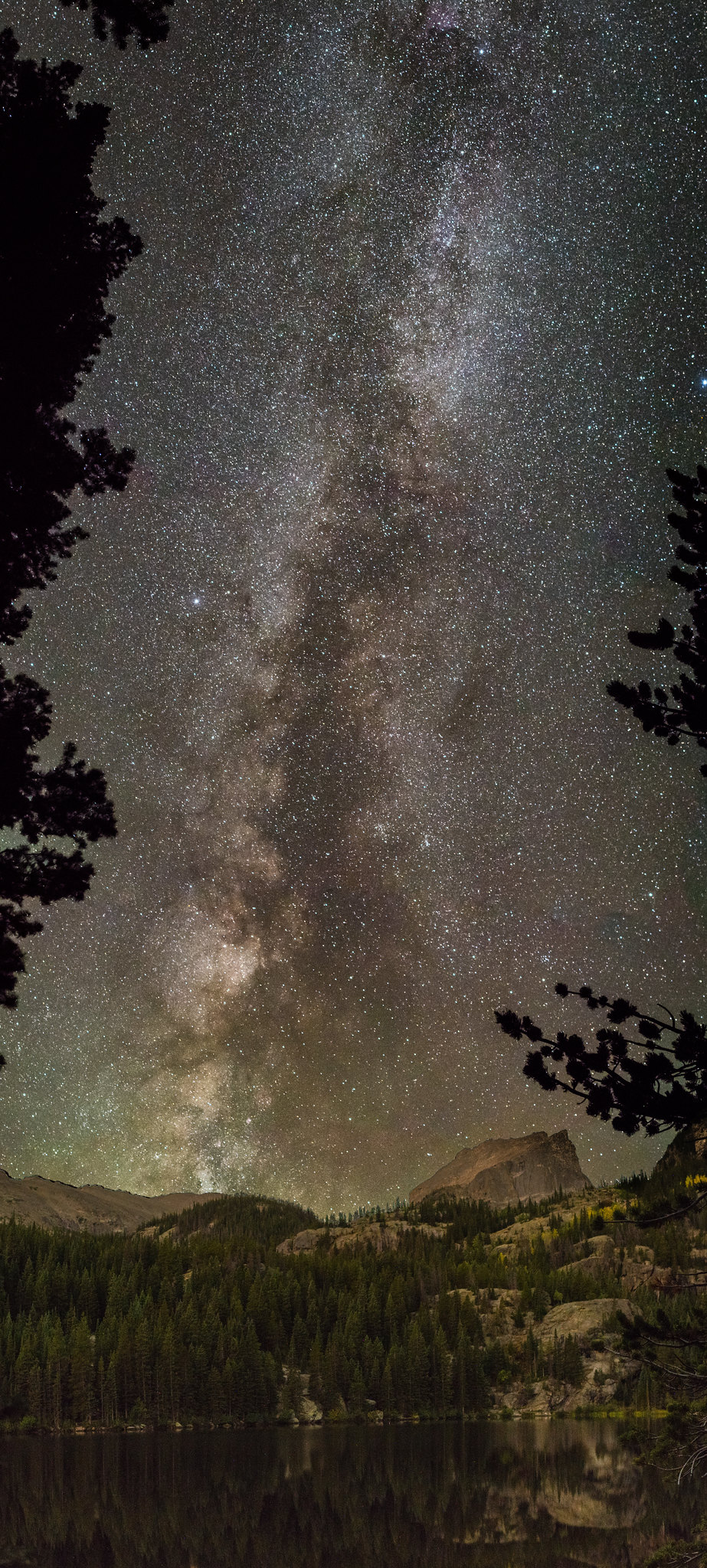The image presents a breathtaking night sky brimming with an innumerable array of stars, creating a celestial tapestry that stretches across the majority of the frame. While the sheer perfection of the scene brings to mind photorealistic artistry, it may very well be a genuine photograph, possibly taken from a region of the world renowned for its clear, starlit nights. Wisps of clouds and mist intermingle with the stars, adding depth and a touch of ethereal beauty to the vast expanse above.

Below this mesmerizing sky, a rugged, mountainous landscape emerges. The rocky terrain ascends gracefully to meet the horizon, its jagged peaks silhouetted against the starry backdrop. The sloping hills give way to dense pockets of trees and lush greenery, cascading down towards the earthy floor of the valley.

Further down, nestled at the foot of this undulating terrain, lies a serene body of water—perhaps a tranquil pond or a placid lake. Its surface remains remarkably calm, mirroring the verdant trees that line its perimeter. The absence of any text in the image allows the viewer to fully immerse themselves in the natural beauty and quiet majesty of this nocturnal scene.